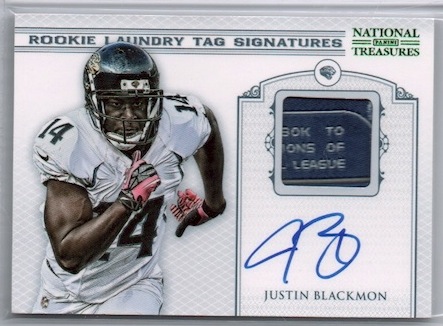This promotional item showcases an African-American football player, Justin Blackmon, in a dynamic running pose. He dons a black helmet and a white uniform emblazoned with the number 14. His attire includes white pants and gloves that feature black, pink, and red elements. Displayed above the player, in a bluish hue, is the text "Rookie Laundry Tag Signatures," while "National Treasures" appears in green on the top right. An incomplete phrase, "Bach II Hons of League," is present, indicating the partial visibility of a larger message. To the right, there is a gravestone-shaped emblem containing a square box, likely representing a part of the laundry tag. Below this, Justin Blackmon's autograph is prominently featured in blue ink. The image radiates a sense of determined athleticism, with the player captured mid-stride, his right arm close to his chest and his left arm extended back. The background is solid white, enhancing the focus on Blackmon and the accompanying text and autograph.